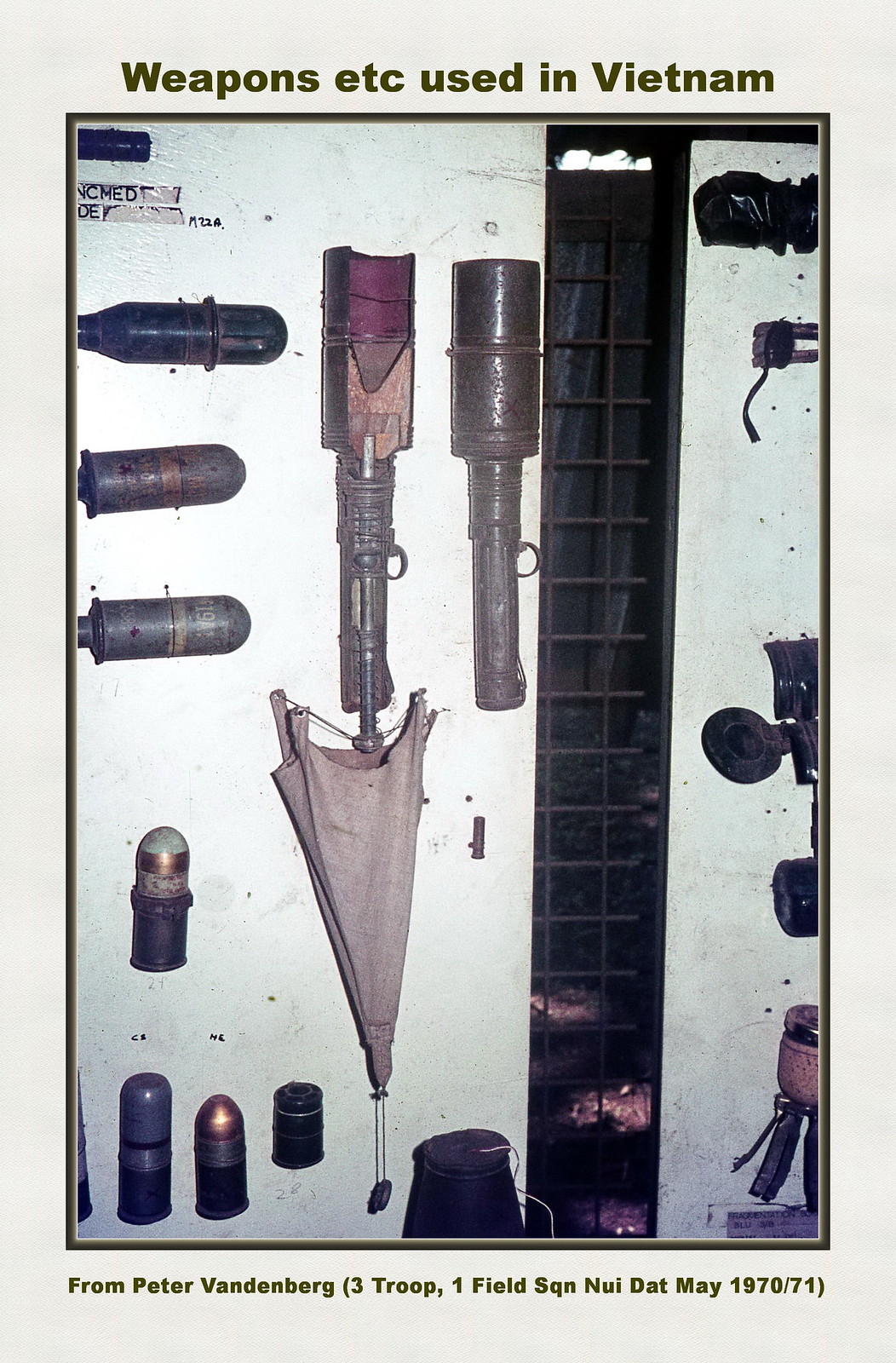The photograph features an array of weapons used in the Vietnam War, all hanging against a wall. The image is framed by two borders: a gray outer border and a thinner dark gray inner border. At the very top, inside the gray border, green text reads "Weapons etc. used in Vietnam." At the bottom, in smaller green text, it says, "From Peter Vanderberg, Troop 3, One Field Squadron, 1970/71." The photograph itself showcases various weaponry, including three cylindrical items with flat ends and bulbous tops towards the left, and two stick grenades with rings to pull on the right. The display is set against a plain wall, and the items appear to be pieces of ammunition or military equipment. Overall, the image is a detailed examination of the kinds of weaponry utilized during the conflict, neatly presented and historically documented.